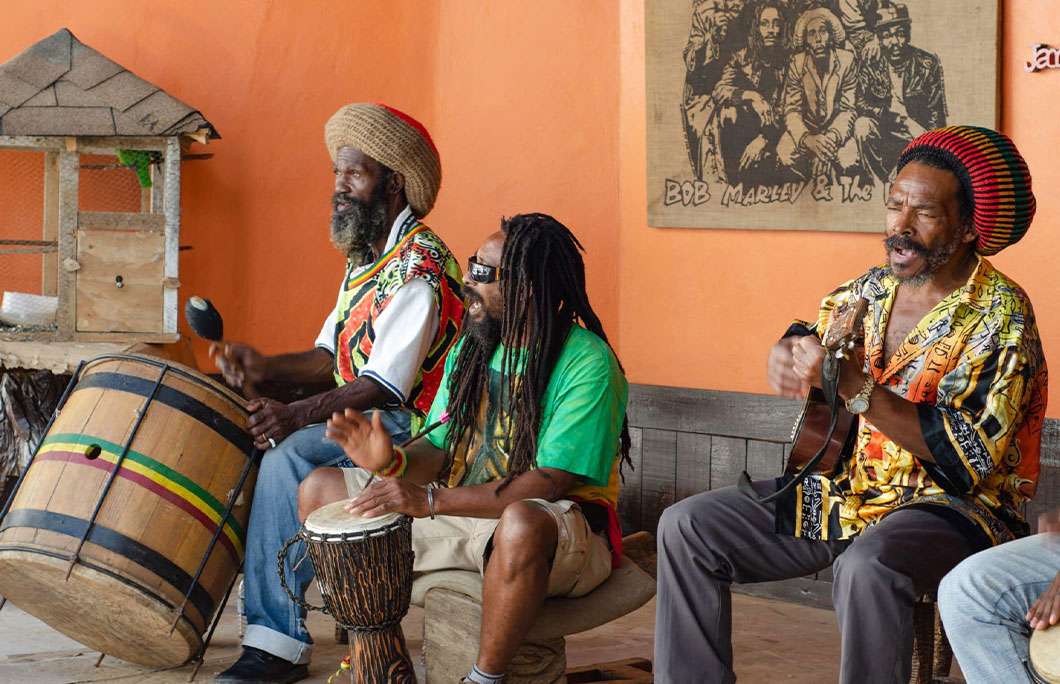In this vibrant outdoor scene, three members of a reggae band sit closely together on a gray bench, immersed in their music. Each musician is adorned in traditional reggae attire, with two of them sporting handmade knit caps likely hiding their dreadlocks, and the other displaying his dreads freely. The man on the left, dressed in a tan cap, commands a large drum emblazoned with Jamaican flag colors. Next to him, the musician in a green t-shirt, sunglasses, and shorts energetically beats a bongo drum. To his left, a third man, clad in a multicolored shirt with shades of orange, black, and red, paired with gray pants, skillfully strums a small guitar, likely a ukulele. 

Behind them, the vibrant orange wall features a nostalgic Bob Marley poster, evoking the spirit and history of reggae. The scene extends to the left where the edge of a wooden and wire bird cage is visible, hinting at the richness of the setting, possibly a cultural venue or market. Additionally, the knee of a fourth unseen person in blue jeans peeks into the frame, adding a sense of casual camaraderie. Nearby, an old cart rests, suggesting it might be used to sell cultural items. The overall atmosphere is one of lively music, cultural richness, and laid-back vibes, harmonizing perfectly with the reggae theme.